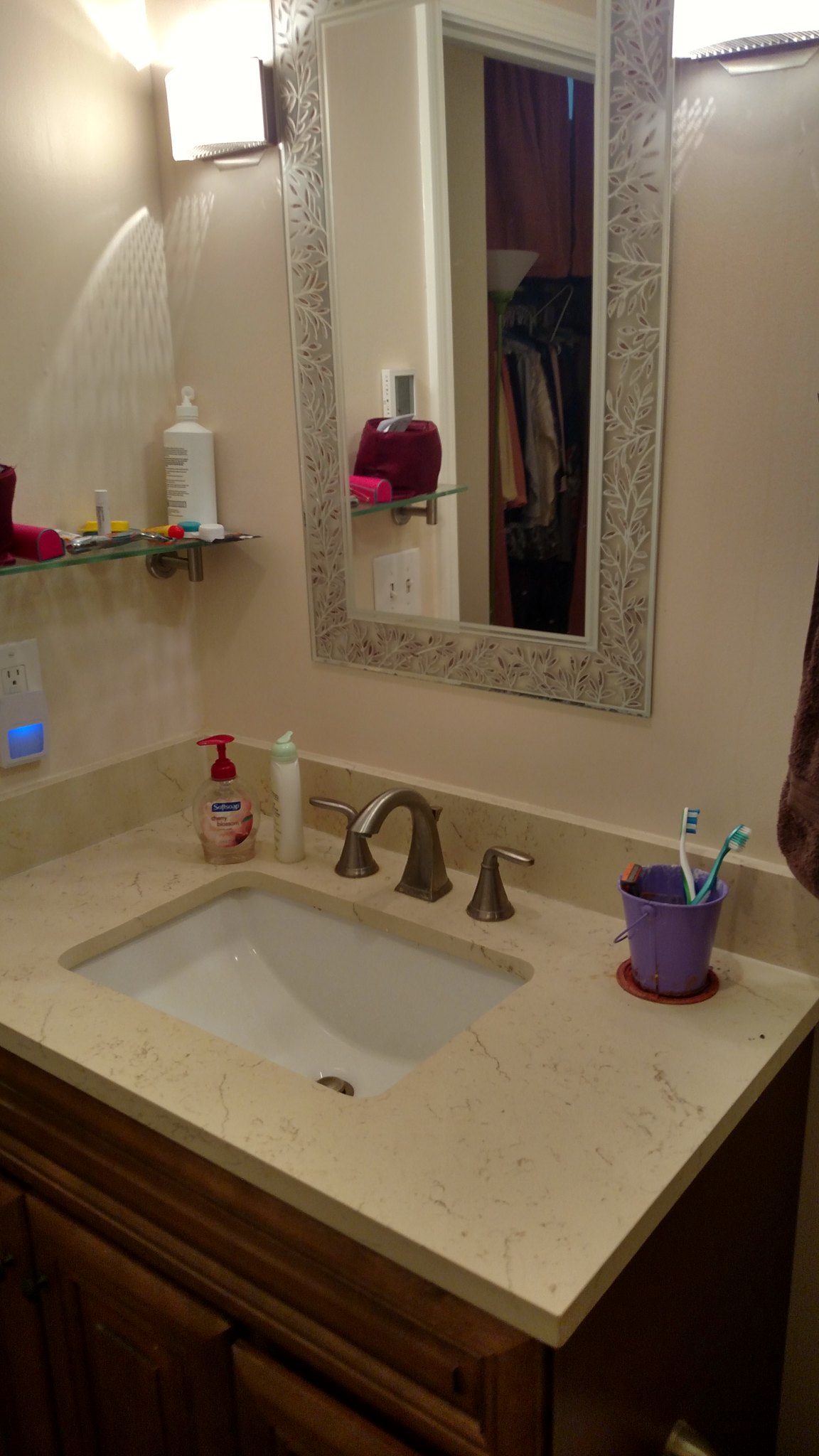The colour photograph, taken in portrait orientation, captures a charming bathroom scene with a focal point on the sink and the vanity beneath it. The sink area is highlighted by an under-mounted white porcelain basin, flanked by dual tap controls on either side of a gracefully curved faucet tap. 

Above the sink, a beautifully framed mirror draws attention, its border adorned with off-white leaves set against a light brown background. The mirror's inner bezel is a sleek, solid silver. The backdrop for this setup consists of faded pink salmon-coloured walls, adding a warm touch to the ambiance.

Adjacent to the mirror, mounted on a wall at a 90-degree angle to the left, is a functional shelf brimming with various items, including bottles and a lipstick pouch. To the right of the sink sits a charming purple toothbrush holder resembling a miniature bucket, complete with a tiny handle on its left side, resting on a red coaster. This holder contains two toothbrushes.

The vanity below features a rich mahogany wooden frame supporting a striking granite countertop. The countertop boasts a yellowish hue with grey speckles, enhancing the bathroom's elegant aesthetic. Just at the edge of the photograph, in the bottom left corner, the top edges of a pair of cupboard doors peek into the frame, suggesting additional storage space beneath the countertop.